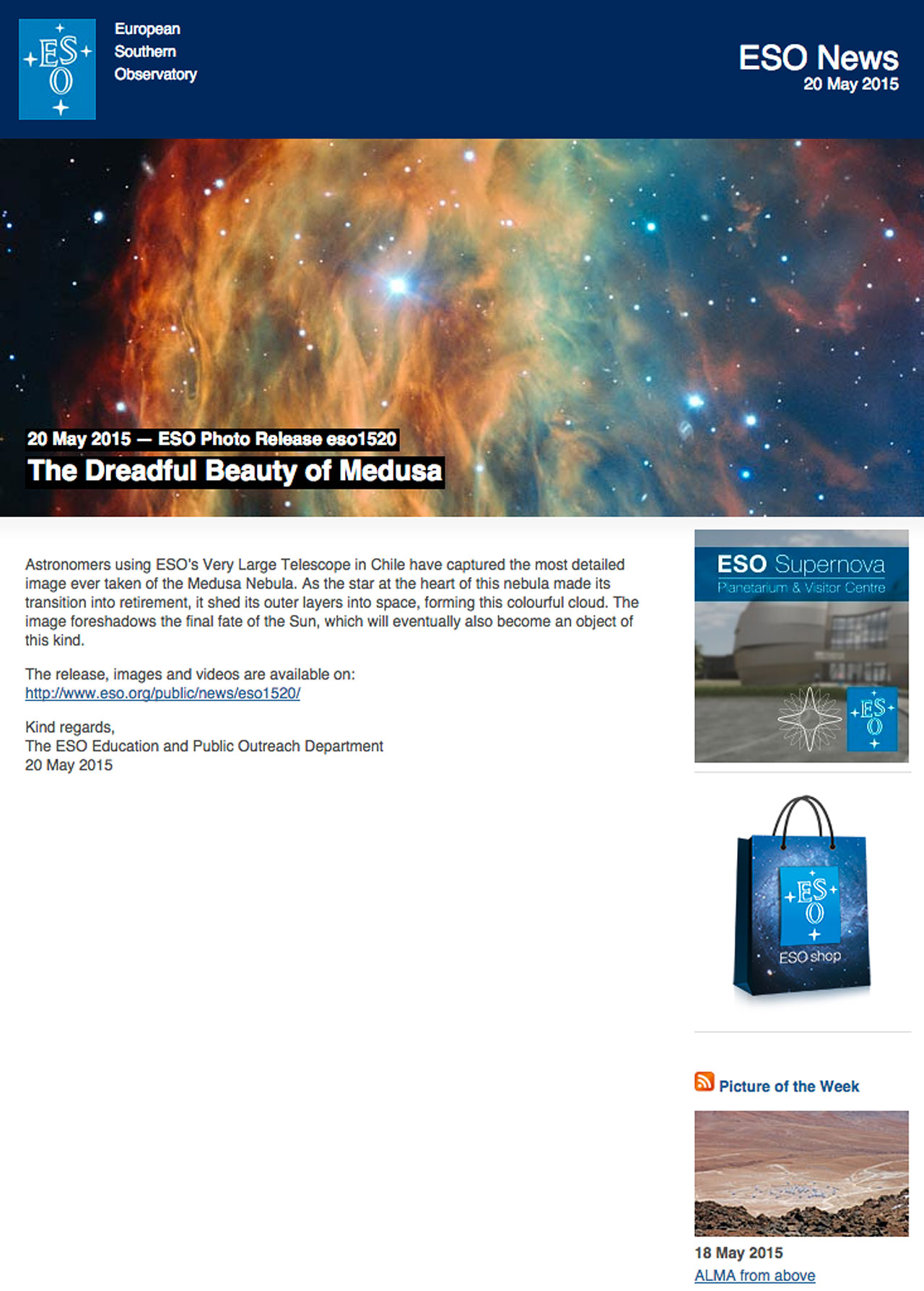This image, taken by the European Southern Observatory (ESO), features an array of notable details. Prominently, the ESO logo and the text "ESO News" are visible, along with a date stamp that reads either May 15, 2015, or May 20, 2015. The caption also mentions an "ESO Photo Release" tag.

On the side of the image, there is a section labeled "Picture of the Week," which appears to show a desert-like landscape accompanied by the title "ALMA from Above." Notably, the letters "A," "L," "M," and "A" are capitalized.

At the top of the image, a building marked "ESO Supernova" can be seen. A detailed description follows, explaining that astronomers using ESO's Very Large Telescope in Chile have captured the most detailed image ever taken of the Medusa Nebula. This image depicts the nebula's central star shedding its outer layers into space as it enters its final life stage, creating a vivid, colorful cloud. This process is noted as a preview of the eventual fate of our own sun. The caption concludes by mentioning that the release image and accompanying videos are available on a specified website.